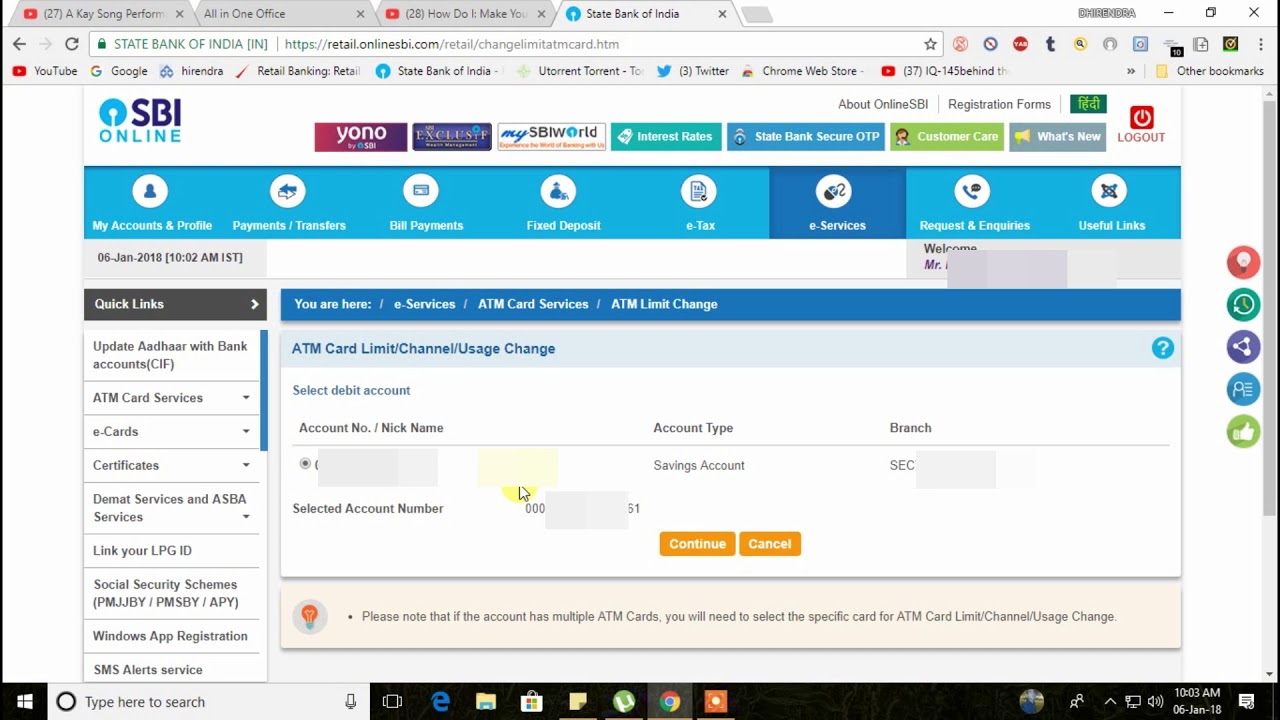Screenshot displaying a webpage titled "SPI Online" viewed in the Microsoft Edge browser. The homepage features a prominent orange button and content related to ATM card loss and usage changes. The layout includes various banner advertisements and navigation menus on the far left side of the screen. On the right, there are multiple social media share icons. The background transitions from white to orange, providing a visually distinct interface. Three browser tabs are open: one for YouTube, another labeled illegibly, and the current tab showing the SPI Online website.